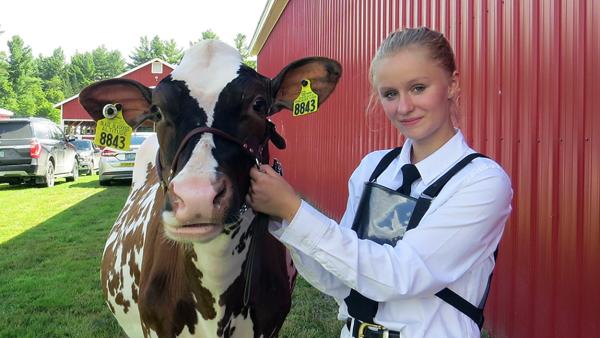This photograph captures a young lady, potentially a teenage girl, during what appears to be a 4-H or county fair animal judging contest. She is standing on a grassy area in front of a large red barn, with additional structures and parked vehicles visible in the background, indicating it is a bright, sunny day in spring or summer.

The young lady is dressed in a white button-down shirt, paired with a black tie, black suspenders or vest, a black belt, and white pants. Her blonde hair is neatly pulled back, giving her a polished and professional appearance. She’s holding the halter of a brown and white Jersey cow with a pink nose and prominent black markings around its eyes. The cow's ears are adorned with yellow tags numbered 8843, and it stands attentively, looking directly at the camera, just like the young lady who has a slight smirk on her face, exuding confidence.

To the left of the frame, green grass and trees add to the vibrant, bucolic atmosphere. The scene vividly captures the essence of rural fairgrounds and the young lady’s participation in livestock showing at a fairs or agricultural event.